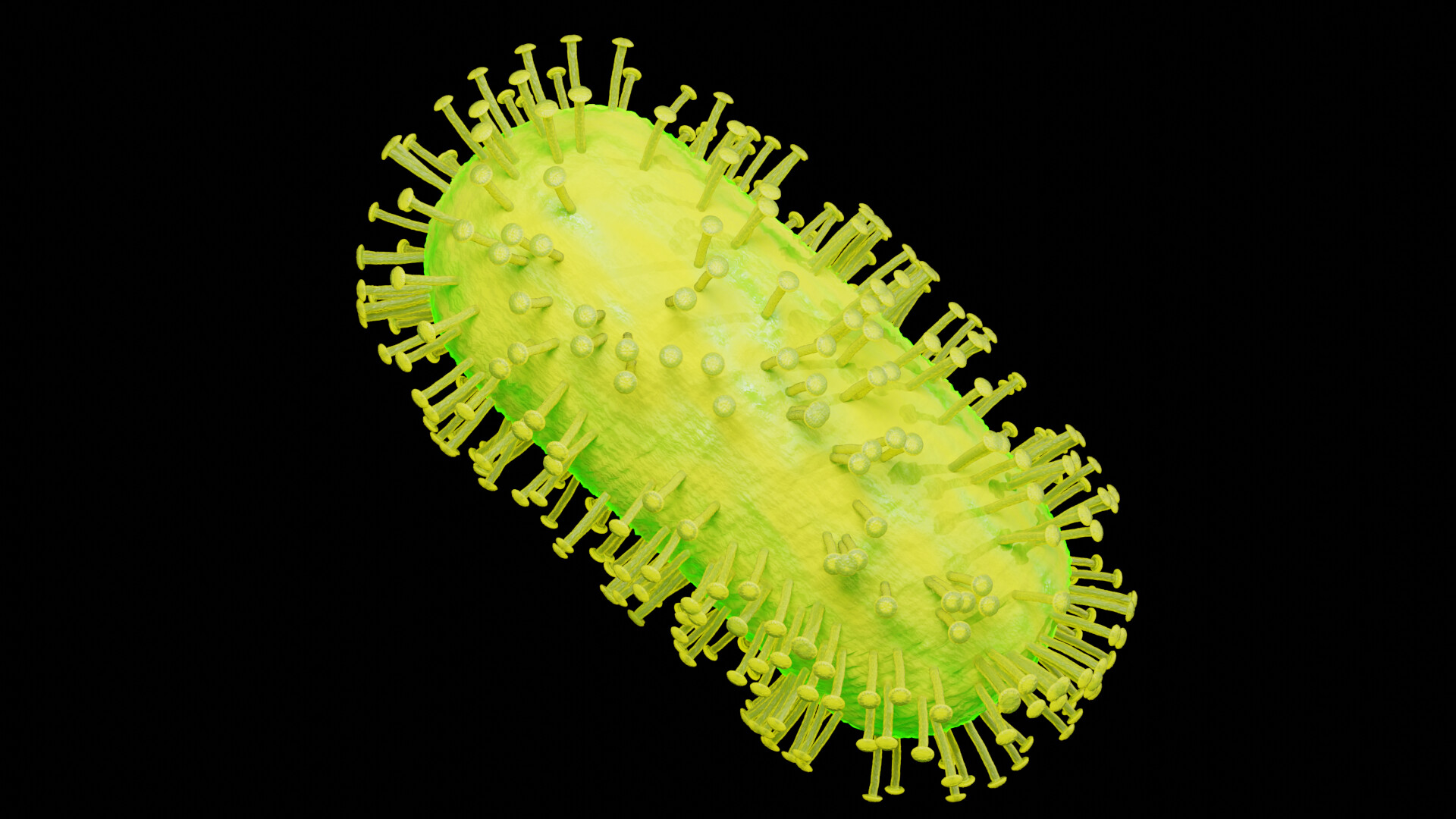The image depicts a detailed artistic representation of a bacterium or germ against a stark black background. Positioned at an angle, from the upper left to the bottom right, the organism has an oblong, tubular, oval-shaped structure with a sickly yellowish-green color that becomes greener toward the borders. The surface of this bacterium is not smooth; rather, it features ridges, lines, and textural details. The most striking characteristic is the numerous spike-like structures, resembling pushpins with some featuring rings around their tips. These structures, varying slightly in appearance, cover the entire bacterium, giving it a densely armored look. This highly detailed drawing or artistic rendition highlights the intricate surface details and the peculiar spike-like protrusions that adorn the organism.